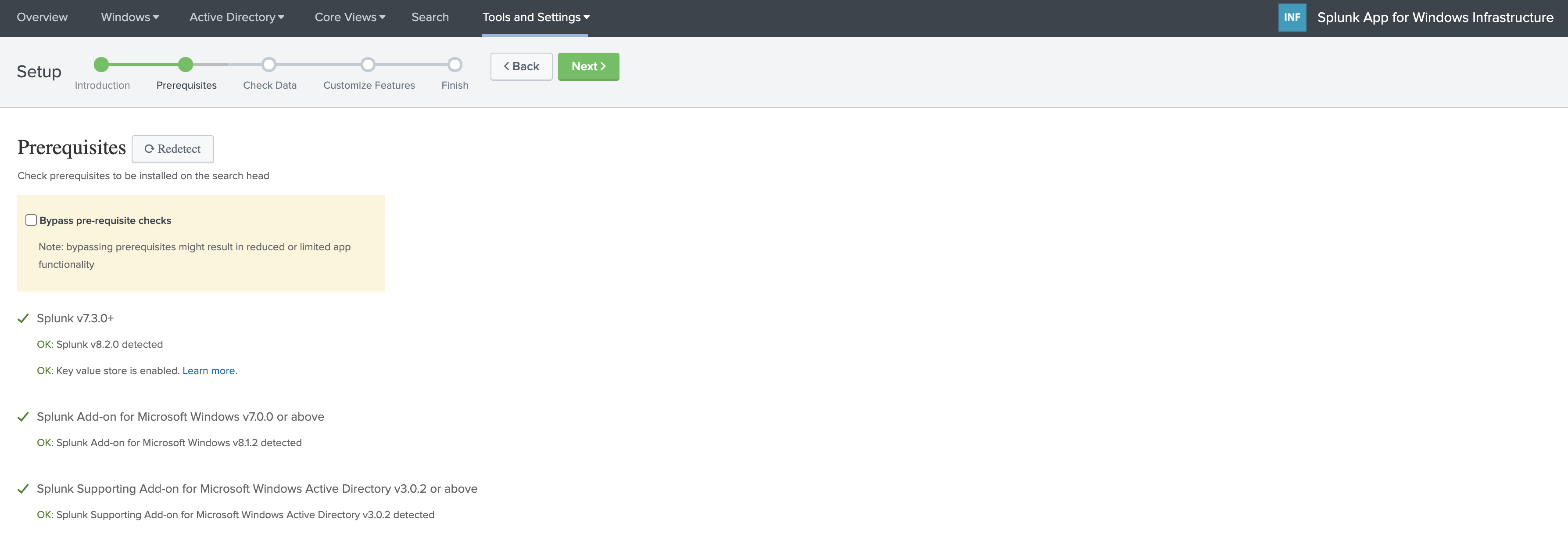This image is a detailed screenshot of the setup process for the Splunk app specifically designed for Windows infrastructure management. The interface is defined by a black navigation banner situated at the top, indicating that it is the Splunk app for Windows infrastructure. This banner contains white text options for navigating different features: Overview, Windows (with a drop-down menu), Active Directory (with a drop-down menu), Core Views (with a drop-down menu), Search, and Tools and Settings (also with a drop-down menu). Currently, the 'Tools and Settings' option is selected, as indicated by a small black line beneath the text.

Directly below the navigation banner, to the left of the screen, there is a progress indicator for the setup process presented as a vertical timeline. The steps are as follows: Introduction, Prerequisites, Check Data, Customize Features, and Finish. The current step highlighted is 'Prerequisites.' To the right of this indicator are navigation buttons: a back arrow and a green 'Next' button, both enclosed in boxes.

The central portion of the screen is dominated by the title 'Prerequisites' in bold, flanked by a 'Redetect' button with a circular arrow icon indicating a reset or redo function. Beneath this heading, there is a small description explaining the check for prerequisites on the search head. This section includes a pale yellow warning box with the option 'Bypass Prerequisite Checks,' which is currently unchecked, cautioning that bypassing these checks could lead to reduced or limited app functionality.

Following this, detailed prerequisite information is listed:

- **Splunk V 7.3.0 Plus**: Indicated as OK in green.
- **Splunk V 8.2.0 Detected**: Also marked OK in green.
- **Key Value Store Enabled**: Includes a 'Learn More' hyperlink next to it.
- **Splunk Add-on for Microsoft Windows V 7.0.0 or above**: Marked OK in green with the specific version detected being **V 8.1.2**.
- **Splunk Supporting Add-on for Microsoft Windows Active Directory V 3.0.2 or above**: Again indicated as OK in green with **V 3.0.2** detected.

No other text or graphical elements are visible within the frame, leaving a clean, concise setup interface.